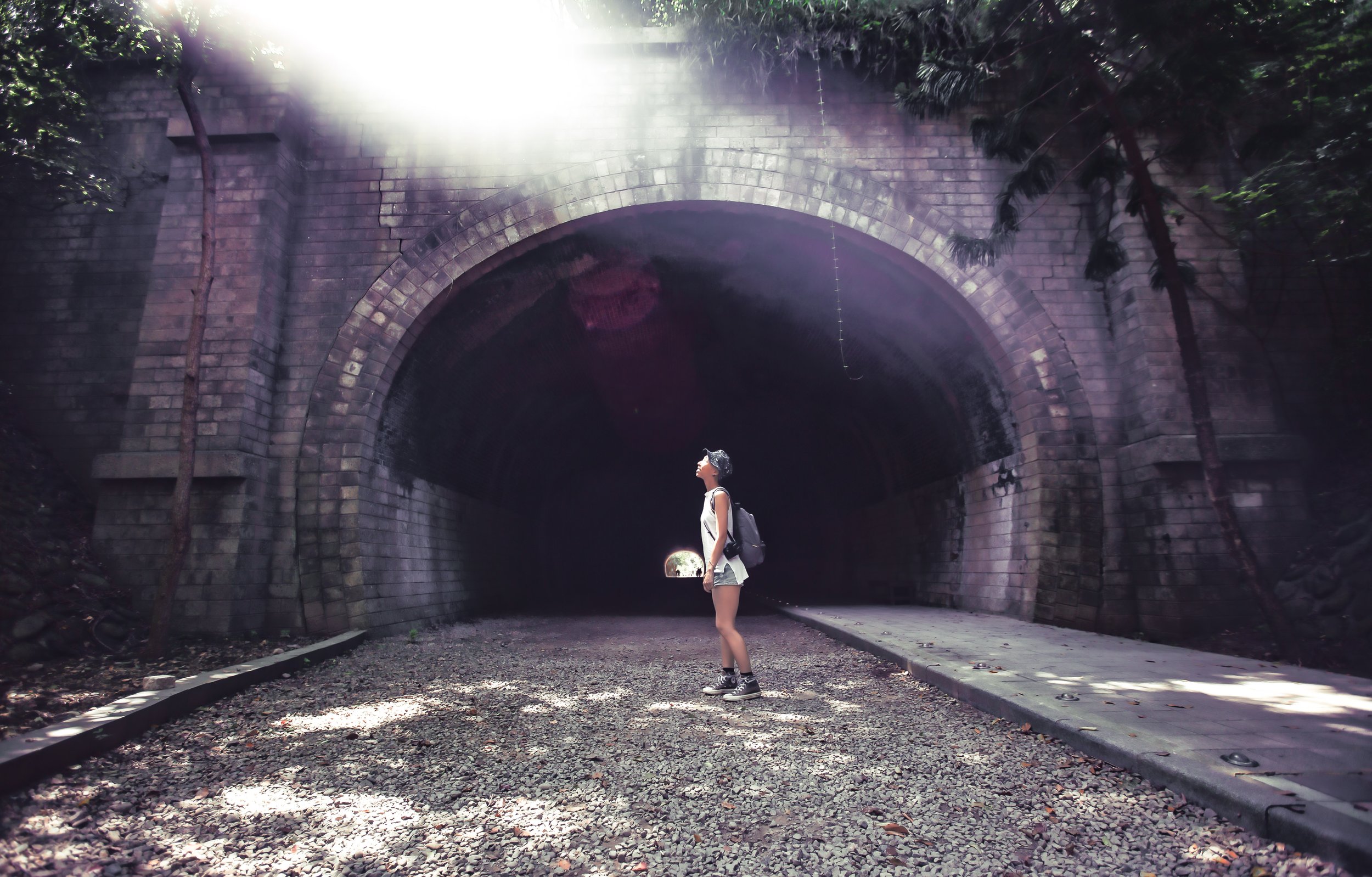In the photograph, the entrance of an old, brick tunnel with a gravel road in front reveals the architectural wear of time. The tunnel is arched with a brick-lined entryway and flanked by rectangular, brick columns on either side. The scene is illuminated by a bright sunbeam streaming from the top left, casting light and shadow play on the gravel path which is intersected by a gray walkway. Trees with leafy branches and vines drape over the walkway, partially shadowing the entrance, which remains dark and mysterious inside.

In the middle of the gravel path, a girl stands, wearing short shorts, high-top black tennis shoes with white soles, and a sleeveless high-neck tank top. Her light brown skin is slightly sunlit as she looks up to the left, possibly towards the sunbeam. She sports a blue baseball cap and a gray backpack, and appears relaxed, holding a tennis racket in one hand. The warmth of the bright day suggests it’s spring or summer, adding to the picturesque yet slightly eerie ambience of the aged tunnel entrance.